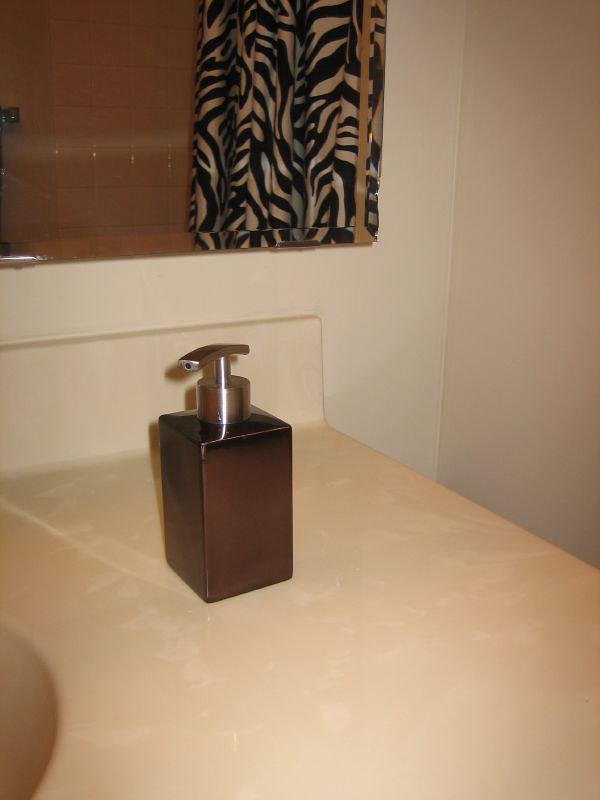The image captures a portion of a bathroom sink area, where the sink itself features an off-white, marbled finish. The surrounding walls are an off-white shade, contributing to a neutral, clean aesthetic. Positioned slightly to the left on the sink is a prominent, square-shaped dispenser—potentially for lotion or soap—distinguished by its brown body and silver top with a matching silver pump. Directly behind the sink, a wall-mounted mirror reflects a shower area adorned with pink tiles. The shower is further accented by a striking zebra-patterned, black-and-white shower curtain. The primary focus of the image is the brown and silver dispenser, which stands out against the understated background.